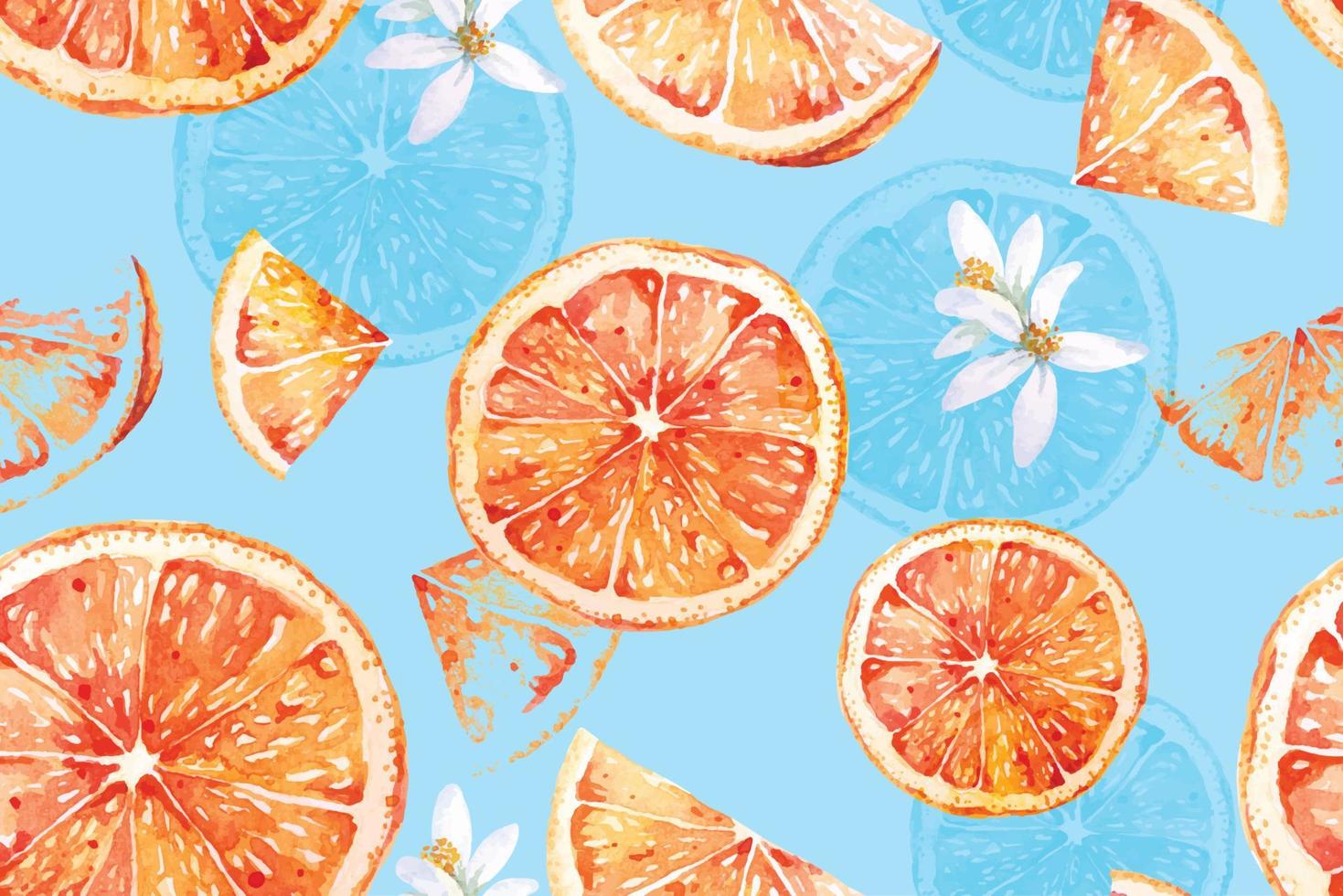The image features a light sky blue background adorned with pale, patterned outlines of halved citrus fruits, arrayed in circular formations showing their internal triangular segments. Superimposed on this backdrop are fully rendered, vibrant, orange slices that display detailed textures: a thin outer skin, an inner whitish rind, and triangular pie-like segments with shiny white specks. Additionally, there are long white-petaled flowers with orange filaments accentuating the image. This detailed and texturally rich depiction, possibly a wallpaper or the front of a card, combines the serene hues of the background with the lively, contrasting colors, and intricate details of oranges and flowers, creating a visually intricate and harmonious composition.